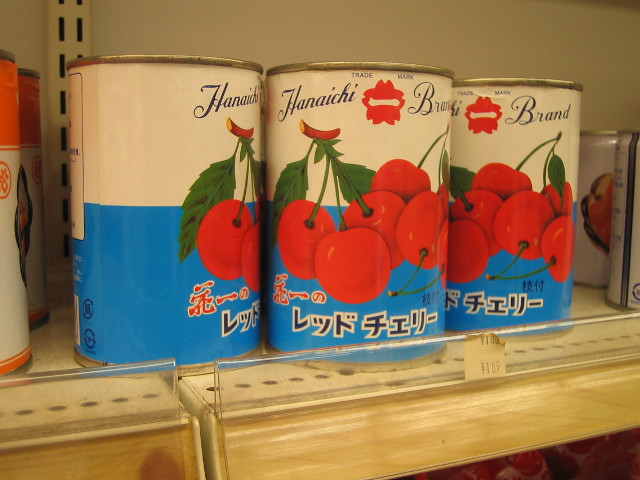The image portrays a can of Hanaichi brand cherries resting on a counter. The label prominently features vivid images of bright red cherries with green stems. The can's design is divided into two sections: the top half is white, while the bottom half is a light blue. The brand name "Hanaichi" appears on the label, written in one of the Japanese alphabets, either Hiragana or Katakana. Between the words "Hanaichi" and "brand," there is a distinctive red emblem, somewhat reminiscent of a star, featuring a white line running through its center, which adds a decorative touch to the label.